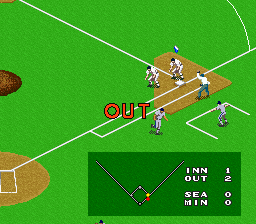This detailed caption describes a screenshot from a baseball video game:

In this still image from a baseball video game, the scene is dominated by a vibrant, grassy green field with the distinct chalk lines of a baseball diamond clearly outlined. Positioned in the center right third of the image are four baseball players. One player has thrown his hat into the air, captured mid-flight against the sky. Meanwhile, two other players are seen running off to the left side of the frame. Prominently, the word "OUT" appears in bold orange text, indicating a game event. In the bottom right corner, a darker green rectangle overlays part of the baseball diamond and contains game score details: "IN ONE, OUT TWO, SEA 0, MIN 0," all written in white text.